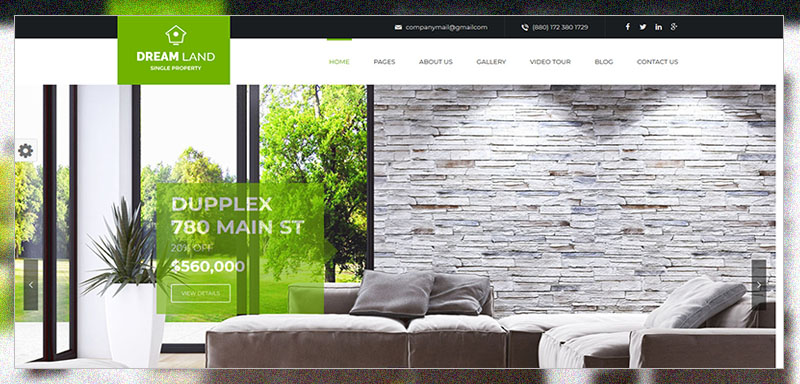This web page showcases the Dreamland Single Property. At the top part of the page, a green rectangle features the title "Dreamland Single Property" in white text, accompanied by a small house icon above it. Directly below, another green square displays crucial property details: "Duplex, 780 Main Street" with a stated price of $560,000 and a mention of "20% off" alongside a "View Details" prompt. This green square overlaps a photo depicting a cozy living room that opens up to a well-maintained green yard with tall, leafy trees. The living room itself boasts an interior with a white brick wall, a large gray sectional sofa, and a potted plant adding a touch of greenery. To the left side of the page, a small gear icon is visible. Above the living room image, there are contact details including an email address, a phone number, and buttons for various social media platforms.